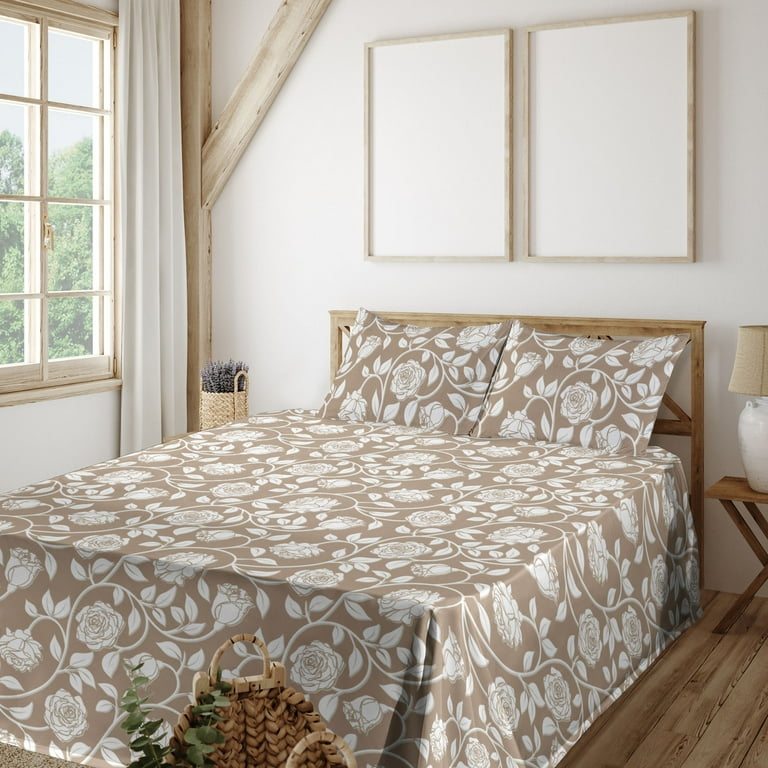The image depicts a well-lit bedroom, characterized by a cohesive and neutral aesthetic dominated by light hardwood flooring and light wood furnishings. The double bed, which prominently features a light brown bedspread adorned with white floral patterns, is paired with matching pillows that are propped against a light wood headboard, seamlessly coordinating with the floor. Above the bed, two solid white paintings with slight brown frames hang on the white wall, contributing to the room’s minimalist decor. On the left side, a window with a light wood frame reveals a view of green trees, suggesting a bright daytime setting, enhanced by the natural light streaming in. A white drape partially covers the window. To the right of the bed stands a wooden nightstand, topped with a white lamp featuring a brown lampshade. In the lower corner, a basket with green stems, and possibly flowers, adds a touch of nature to the room. Additionally, a vertical wooden piece extends from the top to the bottom of the upper left corner of the room, adding a unique structural element. Overall, the room exudes a simple, clean, and somewhat generic feel, reminiscent of a hotel room.